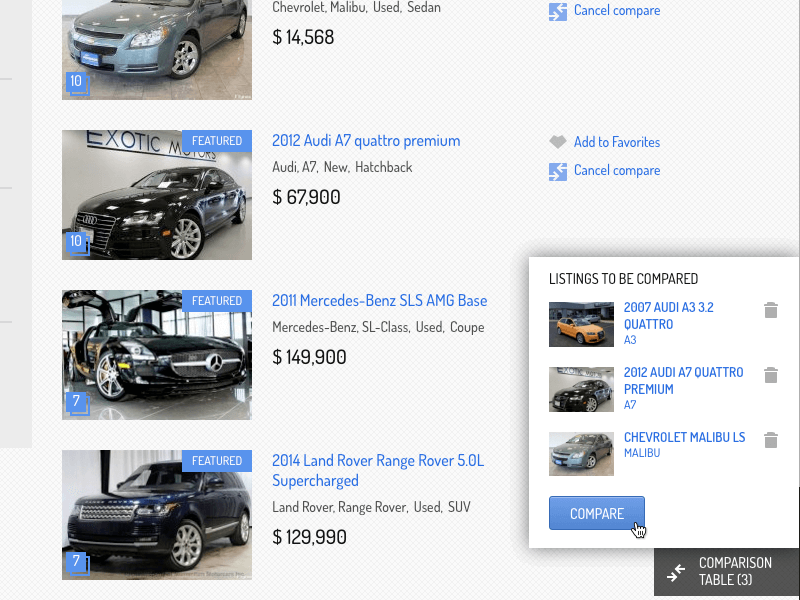This image displays a list of vehicles available for sale. The list includes seven vehicles showcased from top to bottom as follows:

1. **2012 Chevrolet Malibu**
   - Type: Used Sedan
   - Price: $14,568

2. **Audi A7 Quattro Premium (New)**
   - Type: Hatchback
   - Price: $67,900

3. **2001 Mercedes-Benz SLS AMG Base**
   - Type: Used Coupe
   - Price: $149,900

4. **2014 Land Rover Range Rover 5.0L Supercharged**
   - Type: Used SUV
   - Price: $129,990

On the right side of the main section, there's a smaller box containing three vehicles listed for comparison. The text above these vehicles reads "Listings to be Compared." The vehicles in this box are:

1. **2007 Audi A3 3.2 Quattro**
2. **2012 Audi A7 Quattro Premium**
3. **Chevrolet Malibu LS**

A button labeled "Compare" is featured next to these comparison listings, with a hand icon pointing towards it. At the bottom right corner of the page, the words "Comparison Table" are displayed with the numeral "(3)" in parentheses, likely indicating the total number of vehicles selected for comparison.